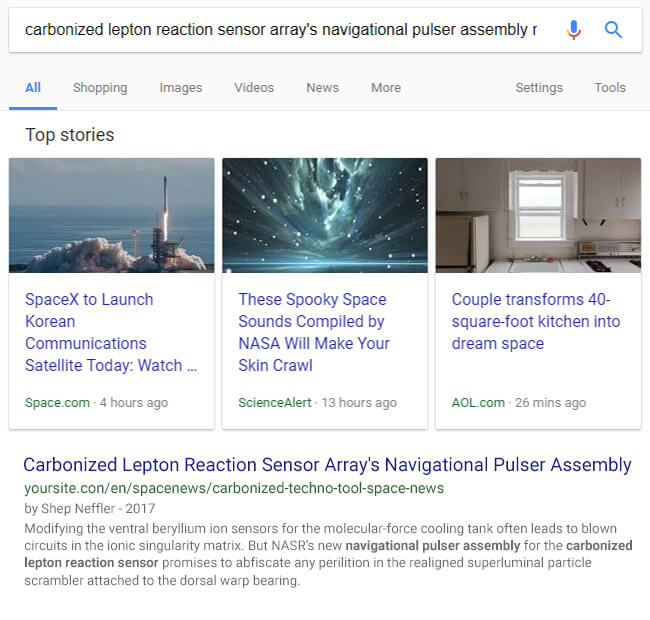In the provided screenshot, a search query has been entered into Google, specifically "carbonized lepton reaction sensors arrays navigational pulsar assembly," although the full query is cut off. The search box, accompanied by a microphone icon for voice searches and a magnifying glass icon, stands prominently. Just below the search box, gray menu options such as 'All', 'Shopping', 'Images', 'Videos', 'News', and 'More' are visible, with 'All' highlighted in blue and underlined to indicate it's selected. To the right of these options are 'Settings' and 'Tools' links.

The webpage has a gray background with darker gray text, except for the blue-highlighted 'All'. Beneath these, the section titled 'Top Stories' presents three images. 

1. The first image is from space.com with the headline "SpaceX to launch Korean communications satellite today – Watch..." and a green link. This article was posted four hours before the screenshot was taken.
2. The second image from ScienceAlert depicts a star-filled sky with a glowing blue ground, featuring the headline "These spooky space sounds compiled by NASA will make your skin crawl". The ScienceAlert link is also green, and the post is 13 hours old.
3. The third image is of a kitchen, accompanying an AOL.com article titled "Couple transforms 40 square foot kitchen into dream space." This article was posted 26 minutes ago as per the screenshot timestamp.

Below the 'Top Stories' section, an article from yoursite.com titled "Carbonized Lepton Reaction Sensors Arrays Navigational Pulsar Assembly" by Shep Neffler (2017) appears. The excerpt reads: "Modifying the ventral delirium ion sensors for the molecular force cooling tank often leads to blown circuits in the ionic singularity matrix, but NASR's new navigational pulsar assembly for the carbonized lepton reaction sensor promises to obfuscate any parallelation in the realigned superluminal particle scrambler attached to the dorsal warp bearing." Key terms 'navigational pulsar assembly' and 'carbonized lepton reaction sensor' are emphasized in bold letters.